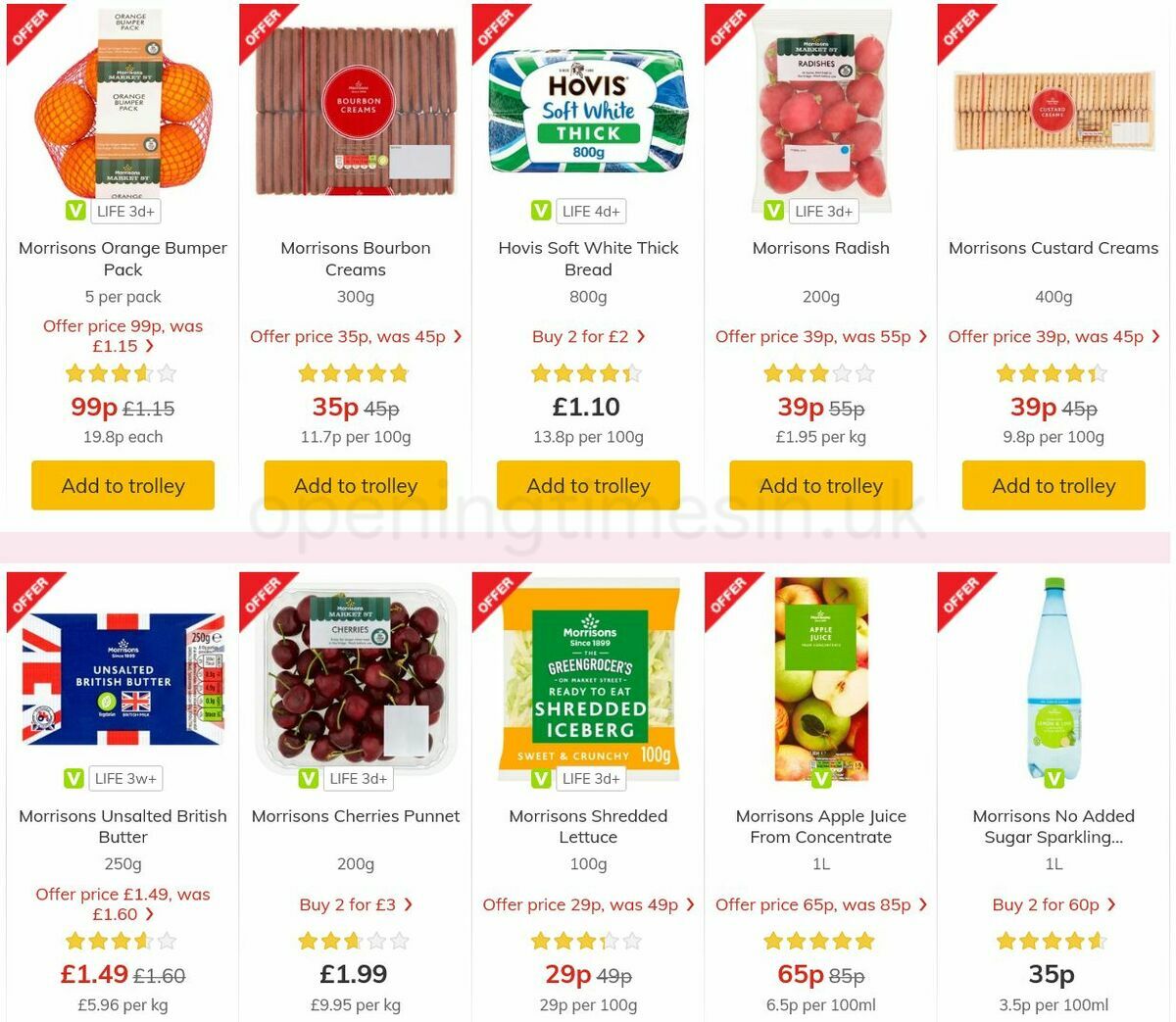A majestic scene captures a solitary mountain peak piercing through a blanket of clouds, with the sun setting in the background, casting a warm, golden hue over the landscape. The play of light and shadow highlights the rugged contours of the mountain, creating a sense of awe and wonder. Below the peak, dense forests stretch across the foothills, gradually fading into the serene expanse of a tranquil lake. The still waters of the lake reflect the surrounding beauty, adding a mirror-like depth to the image. This breathtaking panorama encapsulates the raw, unspoiled beauty of nature.